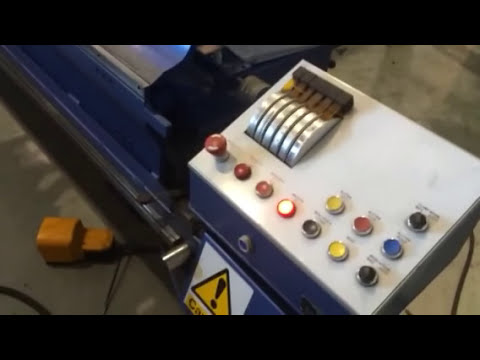This color photograph showcases a control panel for an industrial machine situated within a factory or manufacturing environment. The large, white rectangular control box is centrally featured, adorned with a variety of multicolored push buttons—predominantly red, with some yellow, blue, and black interspersed. Notably, a red button in the middle of the bottom row is illuminated. Above this array of buttons is a small horizontal black box and to the left of it, several silver half-discs are visible. The lower portion of the panel displays a partial view of a warning sign, a yellow triangle with a black border and an exclamation point in the center, cautioning of potential hazards.

Positioned to the left of the control panel is a large orange metal object, resembling a cowbell, lying on the ground. In the upper left section, partially behind the control box, a substantial blue metal object is visible, hinting at more complex machinery. The floor beneath the setup appears to be concrete, with various wires and electrical connections scattered throughout, reinforcing the industrial setting. The overall setup suggests a potentially hazardous environment, as indicated by the cautionary signage.